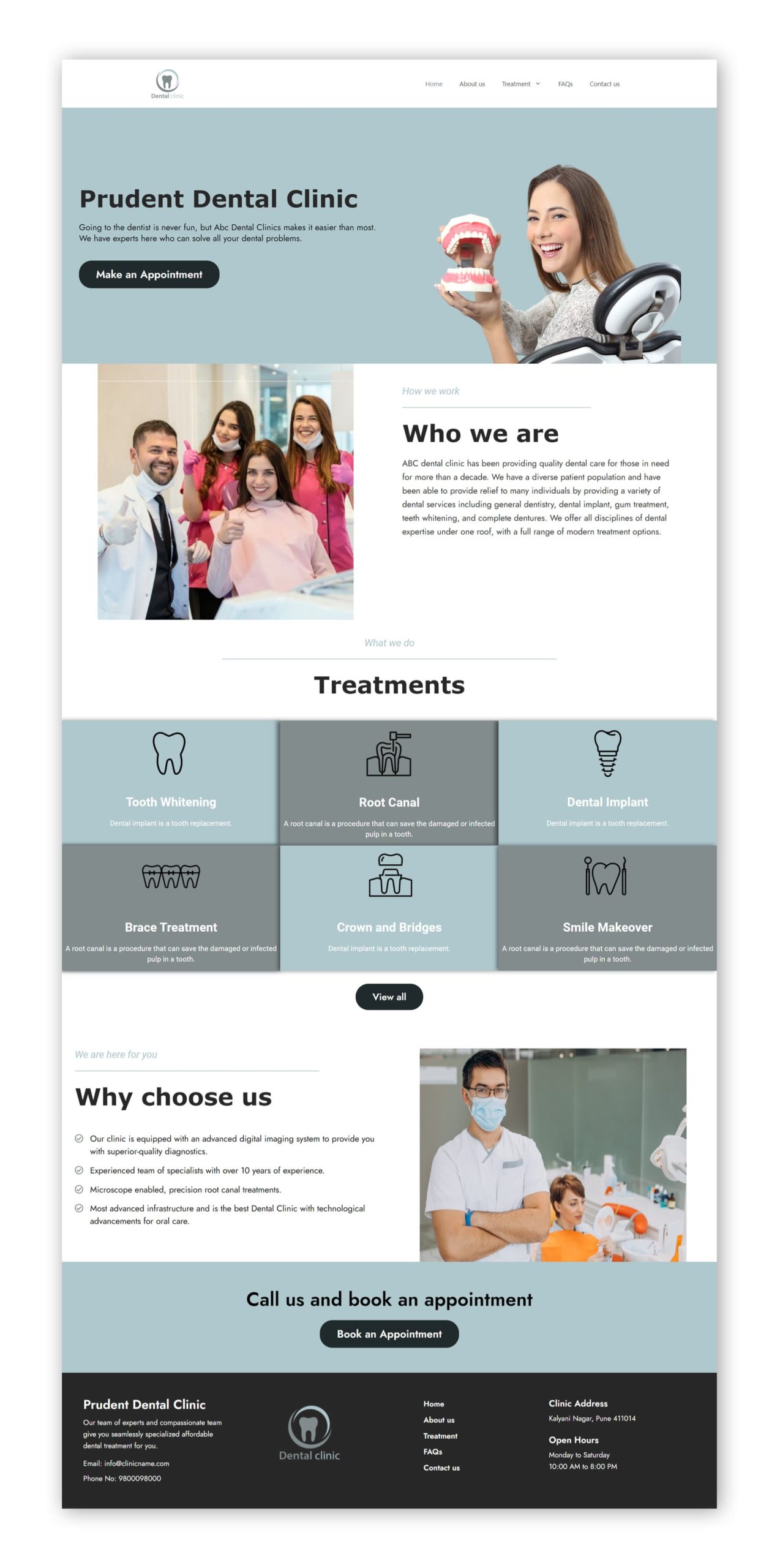The image showcases a detailed view of a dental website named "Prudent Dental Clinic," displayed on a greenish-gray background at the top of the page. On the right side of the homepage, there's an engaging picture of a woman holding both the top and bottom rows of teeth while smiling brightly. To the left, a prominent "Make Appointment" button is positioned. 

Beneath this section, a white block introduces the section titled "Who We Are," featuring photos of the clinic's staff members. Continuing down the page, a section labeled "Treatments" displays icons and descriptions of various services offered, such as tooth whitening, root canals, dental implants, brace treatment, crowns and bridges, and smile makeovers.

Further down, the section "Why Choose Us" presents compelling reasons for selecting the clinic, along with informative content. To the right of this section, there's a picture of one of the dentists, who is wearing a mask and standing with his arms folded. Next to him, a female patient, wearing an orange apron or cover over her clothing, is seated in a dental chair.

At the bottom of the page, there is a call-to-action segment with the text "Call and Book" and "Call us and book an appointment," accompanied by another "Book Appointment" button to encourage visitor engagement.